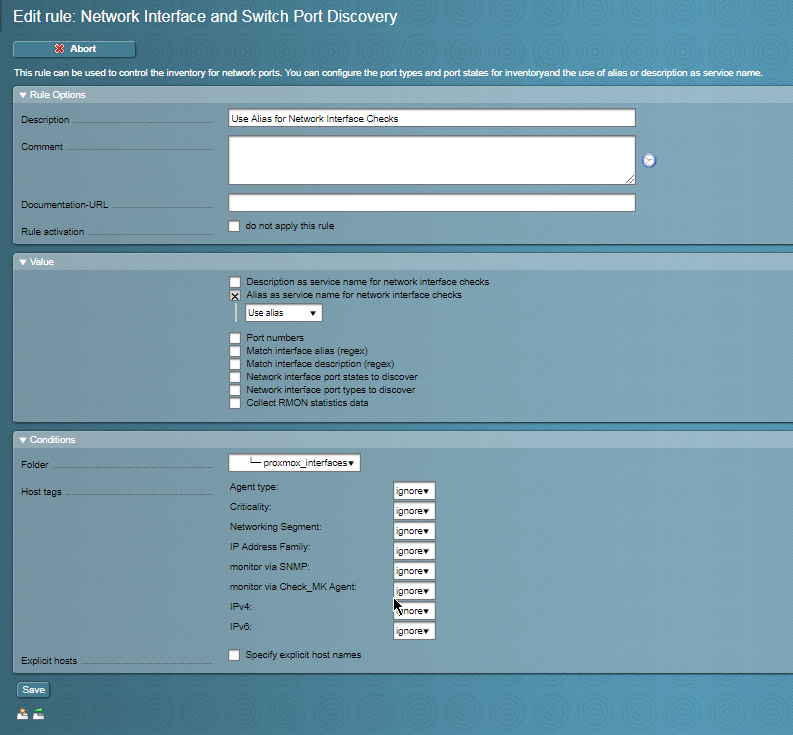The image displays a user interface page with a light bluish-gray background featuring white text at the top that reads, "Edit Rule: Network Interface and Switch Port Discovery." Below this title, there is a red button labeled "Abort" accompanied by a red X icon. The text beneath the button explains that the rule can be used to manage the inventory of network ports, allowing users to configure port types and states for inventory purposes and to use aliases or descriptions as service names.

The interface comprises several sections and boxes: 
1. **Rule Options:** This section includes fields for entering a description, using aliases for network interface checks, commenting, adding a documentation URL, and setting rule activation parameters. There is also a checkbox option titled "Do not apply this rule."
2. **Value:** This part allows users to specify descriptions as service names for network interface checks and to choose whether to use an alias for this purpose, with options that include port numbers, matching interface aliases, or descriptions.
3. **Network Interface Port Settings:** Users can define port states and types for discovery, and choose to collect RMON statistical data.
4. **Conditions:** This final box contains settings for folders, host tags, agent types, critical network segments, IP address families, and monitoring preferences (including SNMP and Check MK Agent). It includes options for both IPv4 and IPv6 and allows the specification of explicit host names.

Overall, the page provides comprehensive tools for configuring and managing network interface and switch port discovery rules.